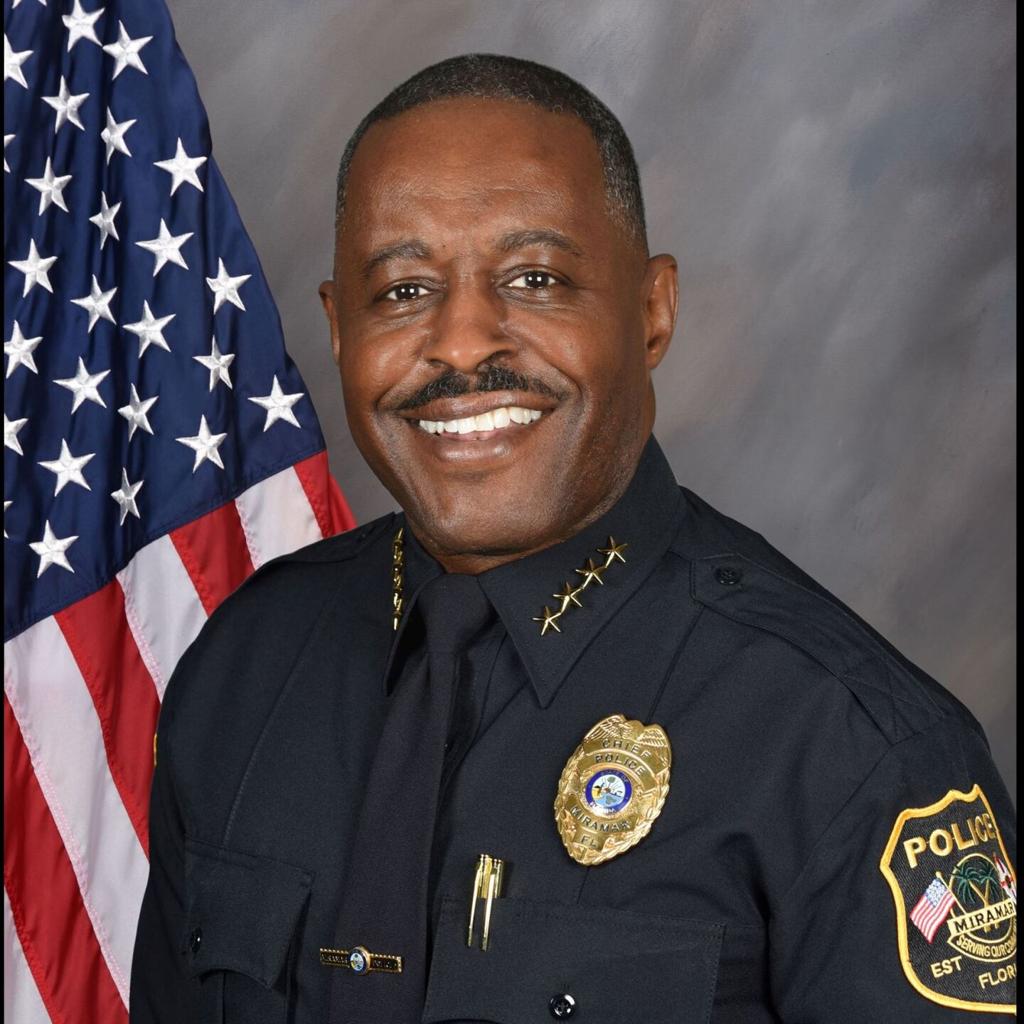This is a highly detailed color portrait of a distinguished African American male police officer in full uniform, standing next to an American flag with a mottled gray backdrop. The officer, who has salt-and-pepper short hair and a mustache, is smiling warmly at the camera. His uniform features four gold stars on each collar, indicating a high rank. He is wearing a black shirt with a tie, which has a golden pin. His name tag and two gold pens are situated above the right breast pocket. The badge on his left chest, with the inscription "Chief Police Miramar, Florida," includes an icon in the center. Additionally, a patch that says "Police Miramar, Serving Our" is visible on his left sleeve, although partially obscured. The overall presentation, along with his professional demeanor and the American flag, suggests this image might be used for official purposes on a law enforcement website.